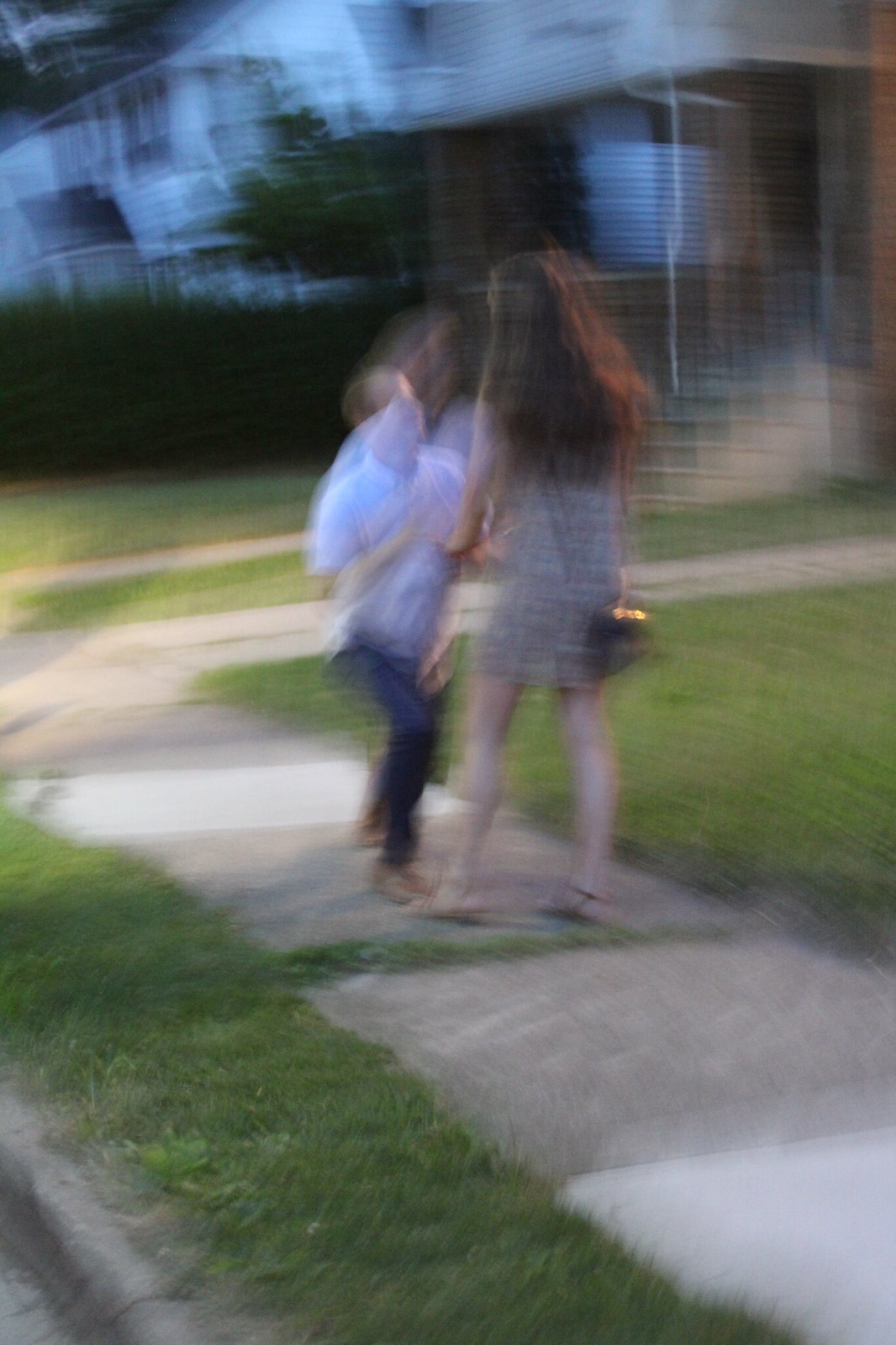This image captures a very blurry scene on a neatly manicured suburban sidewalk, depicting a significant moment between two people. The taller individual, a woman with long brunette hair, stands with her back to the camera, wearing a brown dress that falls above her knees and sandals on her feet. She carries a metallic-colored purse slung on her back. In front of her, a shorter man is caught in a dynamic motion, seemingly in the act of kneeling down, adding a sense of urgency and emotion to the scene. The man, characterized by his receding hairline, wears a white collared short-sleeved shirt, dark pants, and light brown shoes. The sidewalk, marked by visible expansion lines, is flanked by a well-kept lawn on both sides with patches of grass extending towards the curb. In the background, the scene is illuminated by a yellowish light emanating from one of the two-story suburban homes, which are predominantly white with porches, steps, and some surrounding shrubbery and trees, further enhancing the intimate, suburban atmosphere of the early evening.